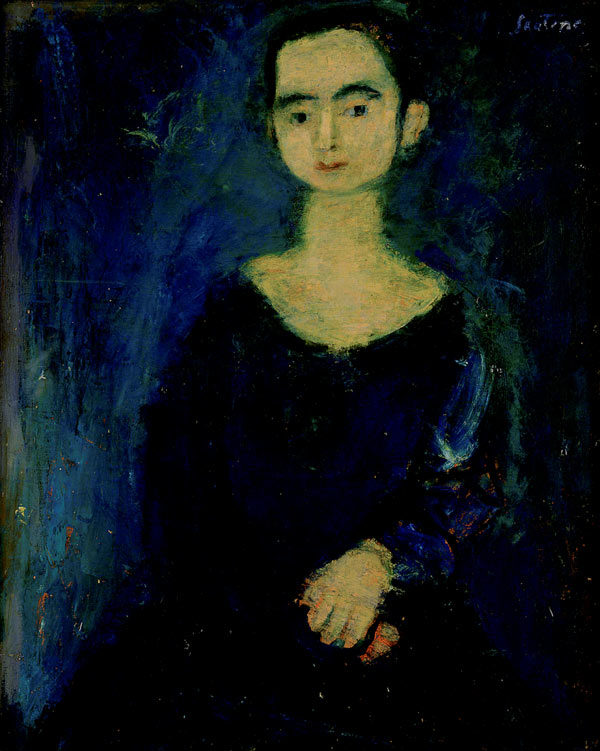The painting portrays a young woman, possibly in a post-impressionist style, rendered in rich acrylic hues dominated by dark blues, blacks, and subtle accents of red and green. She has fair to olive-toned skin, with dark black hair that seems tied back, and expressive, wide black eyebrows above slightly cross-eyed beady black eyes. Her lips are pursed in a thin line of red lipstick, with her right ear sticking out prominently while the left is obscured. Wearing a striking dark blue dress, she sits with her arms crossed on her lap—the left hand covering most of the right hand. The backdrop transitions from a lighter blue around her form, emphasizing a sense of light, to near-black at the edges, creating depth and contrast. The painting includes the artist’s signature at the top right, though it's unreadable.